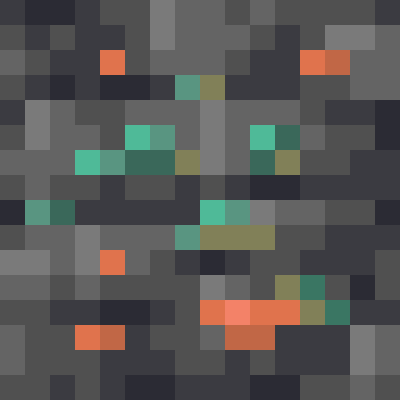The image is a highly pixelated, computerized picture composed of large, square pixels. The primary color represented is gray, encompassing a range of shades from light gray to charcoal, which is just shy of black. Interspersed among the gray tones are various colored pixels: shades of green ranging from pure dark green to light green and olive, as well as shades of orange, from typical orange to more muted, peachy hues. The orange pixels are fewer in number compared to the gray and green squares, while the rarest color featured in the image is the olive green. The overall composition is dominated by the grayscale, giving the image a predominantly monochromatic appearance with occasional bursts of color.